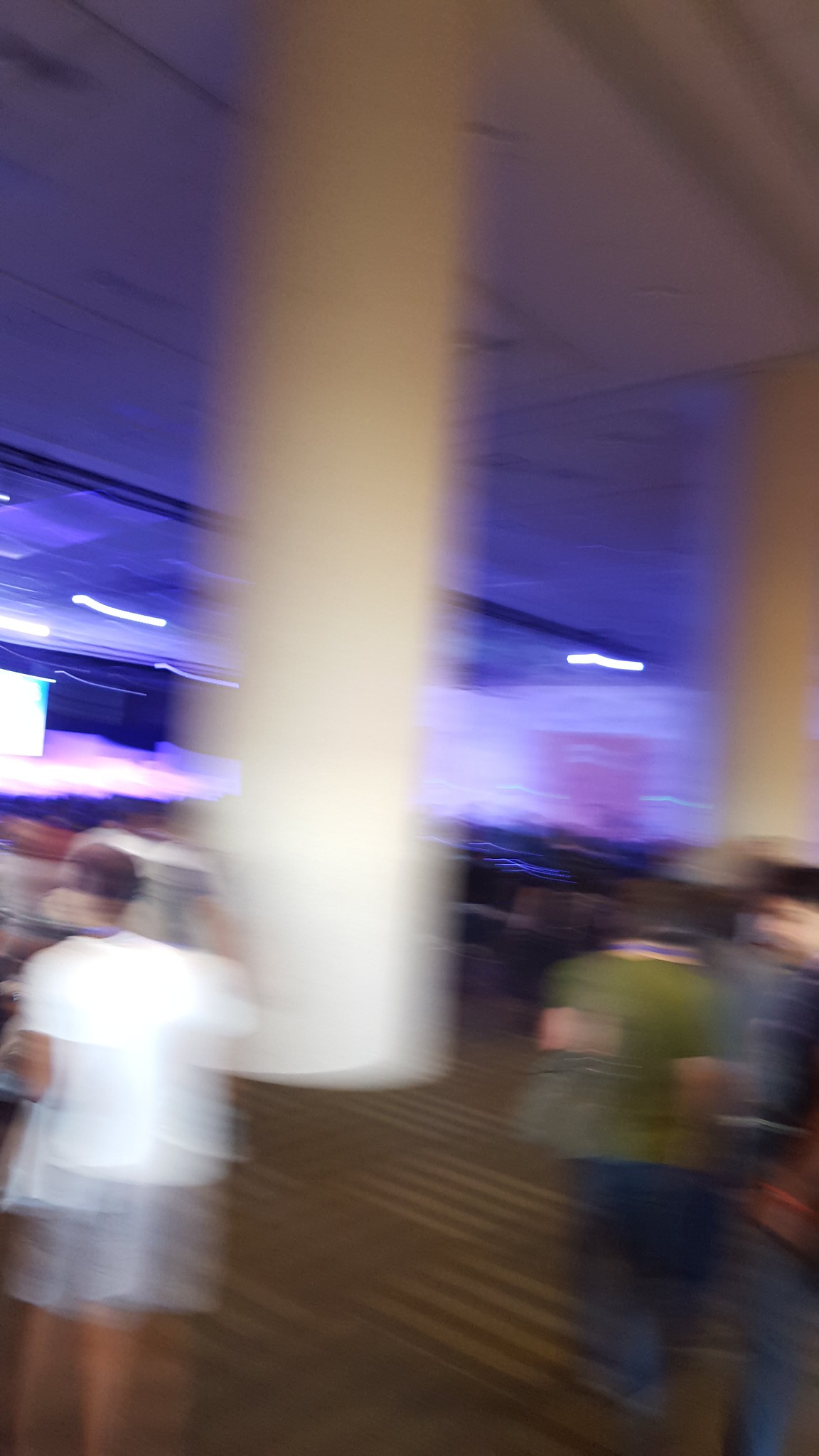A very blurry image of an interior space featuring a central white pillar under an intricately designed ceiling adorned with various types of lighting, including pervasive blue and a distinct purple light at the center. The floor is carpeted. In the bottom left corner, a white shirt and green shirt are visible among blue pants and shorts. The surroundings include several items of furniture and blinds that appear to descend to the ground.